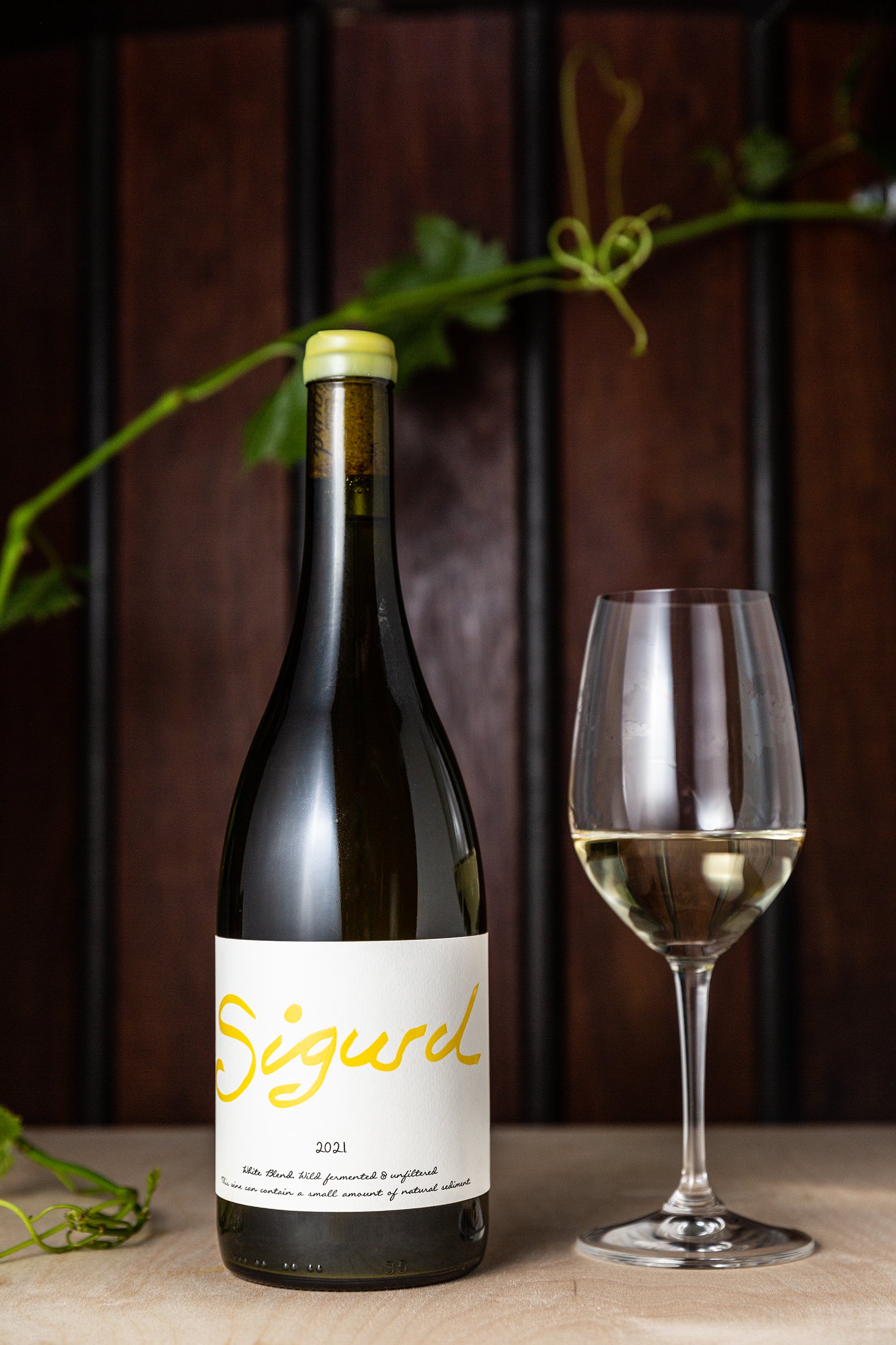A beautifully composed product portrait showcases a bottle of Sigurd wine and a partially filled wine glass, both positioned on a wooden countertop. The wine bottle, capped with yellow wax over a cork, features a distinctive white label with the brand name "Sigurd" written in yellow font. Below, in small black cursive, it reads "2021, white blend, wild fermented and unfiltered," hinting at the bottle’s vineyard origins. The dark glass bottle contrasts subtly with its yellow cap and the white label. To the right, a wine glass filled about halfway with a pale yellow-white wine complements the bottle. The backdrop is a rich, dark cherry wood-paneled wall adorned with a single green vine, possibly a grapevine, which elegantly drapes down and partially rests in the lower left-hand corner of the scene. This setting suggests a rustic, bar-like atmosphere, enhancing the visual appeal of the wine and its natural ambiance.